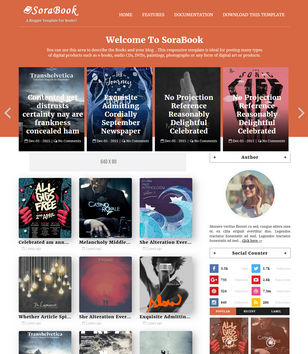The image showcases a screenshot of a book application named "SoraBook". The app's name, "SoraBook", is elegantly displayed in flowing script in the upper left-hand corner, accompanied by a book icon to its left as part of its logo. Beneath the logo, there appears to be a tagline, albeit unclear.

To the right of the logo, there are four navigational options: "Home," "Features," "Documentation," and "Download This Template". Below these options, the app greets users with a welcoming message: "Welcome to SoraBook".

Under the greeting, there's a paragraph of descriptive text. Further down, there is a visually engaging carousel, containing four different graphic items, navigable via left and right arrows positioned on each side of the carousel. 

Below the carousel is a series of thumbnail images, each depicting various graphic items. Among them, one thumbnail clearly reads "All Gigs Free," while another displays "Casino Royale".

On the right side of the app interface, there is a section dedicated to social sharing, allowing users to tag and share the page on platforms like Facebook, Twitter, and other social media networks.

Above the main carousel, there is also a secondary carousel or selection panel that enables users to filter content by author.